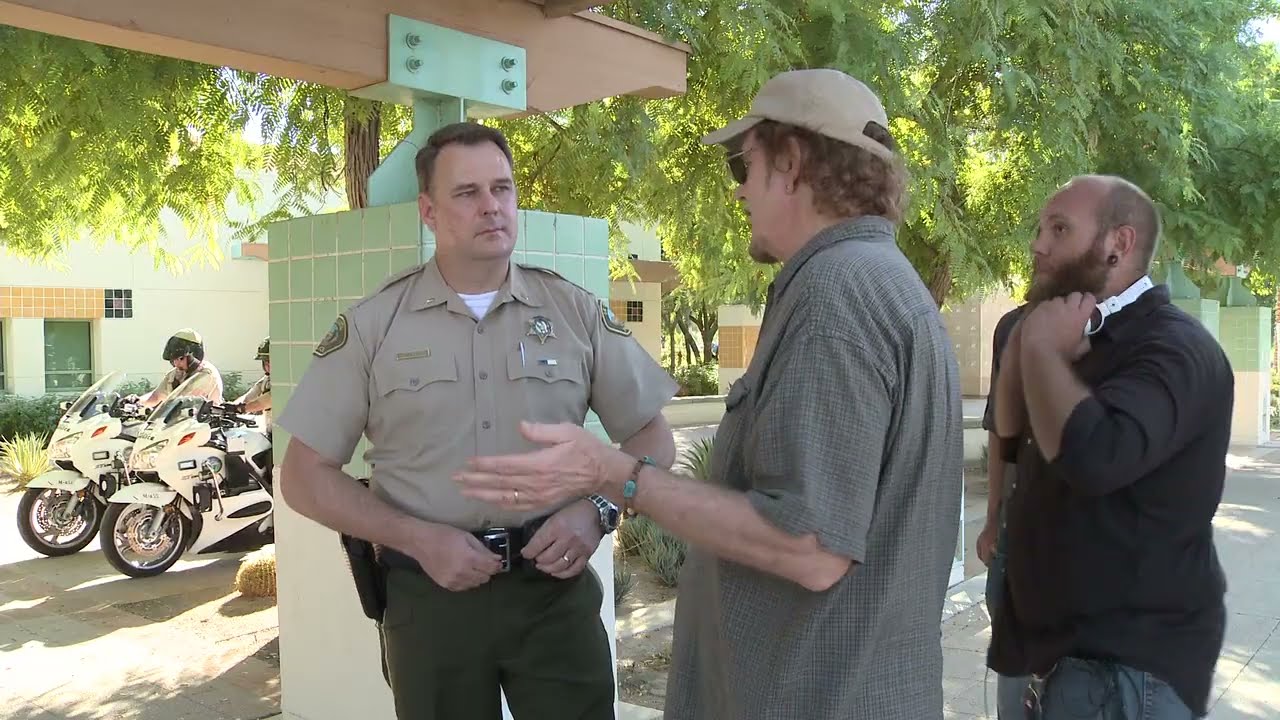The photo features two men standing in front of a white SUV with yellow security lights on top, parked along what seems to be the entrance of a mall or similar building. The SUV, marked with a "9-1-1" sticker and a police department logo, has its driver's side door open. A policeman, identifiable by his olive/tan short-sleeve shirt, olive pants, sunglasses, and a badge, appears to be motioning with his left hand. Adjacent to him is a man in a brown shirt, brown shorts, a cap, and sunglasses, possibly an animal control officer, holding a clipboard. The vehicle is positioned against a backdrop of an entranceway with wood paneling, two tiled pillars, and a shaded overhang, flanked by green leafy trees on either side.